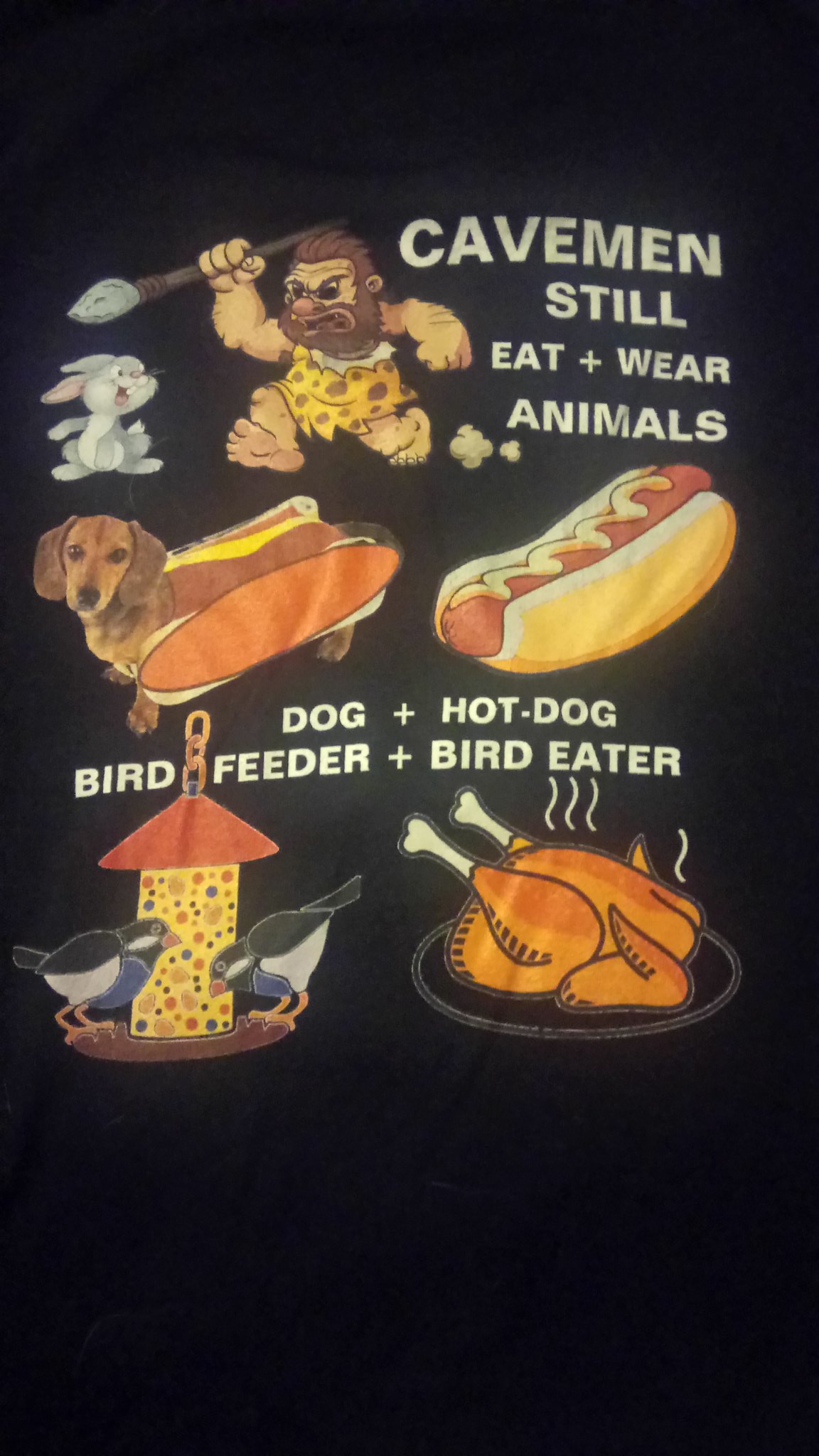The image, set against a black background, resembles a poster or a t-shirt front featuring a series of whimsical cartoon illustrations. At the top, a caveman dressed in a leopard-spotted outfit wields a spear, aiming at a cute rabbit. Accompanying this scene is the text, "cavemen still eat and wear animals." Below, the focus shifts to a humorous depiction of a dachshund dog nestled inside a hot dog bun with a strip of mustard on its back, juxtaposed with a regular hot dog in a bun with mustard. Beside these, the text reads, "dog + hot dog." Moving downwards, the imagery includes a colorful bird feeder with two birds perched on it, labeled "bird feeder," followed by a cooked turkey on a dinner plate, tagged "bird eater."